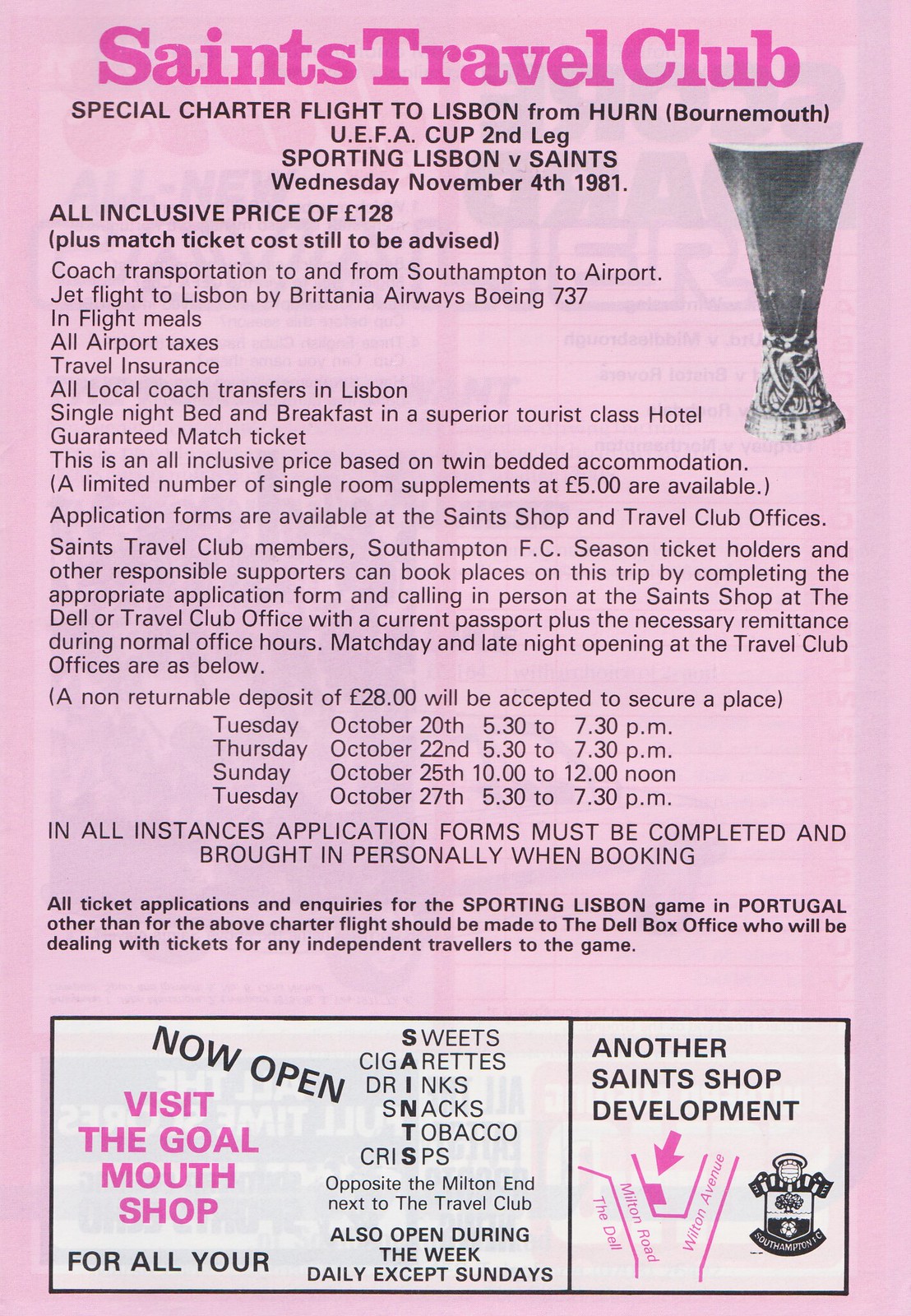The full-page advertisement, set against a very light pink background, announces a special offer from the Saints Travel Club. At the top, bold dark text declares "Saints Travel Club," followed by an all-uppercase announcement, "Special Charter Flight to Lisbon from HURN (Bournemouth) – UEFA Cup Second Leg – Sporting Lisbon vs. Saints – Wednesday, November 4th, 1981." 

To the right of this main heading, there is a photograph of a trophy with an ornate base, while on the left and center of the page, a long block of text provides further details, albeit mostly too small to read. A subheadline reveals an "All-Inclusive Price of 128 Pounds (plus match ticket, cost still to be advised)." This section elaborates on the inclusivity of meals, taxes, coach transfers, and the guarantee of a match ticket, specifically highlighting twin-bedded accommodation.

Centered below the text block, a presumably detailed itinerary or schedule is mentioned, but again, the specifics are too small to discern. Further down, a statement in all caps emphasizes the need for application forms to be completed and brought in personally when booking. Another bold paragraph, too small to read, appears below.

At the bottom of the page, an advertisement is divided into two sections by a vertical black line. The left two-thirds feature a notification for the "Goal Mouth Shop," with the phrase "visit the Goal Mouth Shop" in pink text. Under it, slanted black text proclaims "NOW OPEN," followed by a list offering "sweets, cigarettes, drinks, snacks, tobacco, crisps." Beneath this list, there's additional bold text stating, "Also open during the week, daily except Sundays."

The right third of the ad, with a white background, displays "ANOTHER SAINTS SHOP DEVELOPMENT" in all caps, beneath which is a pink map with a bold arrow pointing leftward and downward, accompanied by an unclear logo or insignia, likely representing the team.